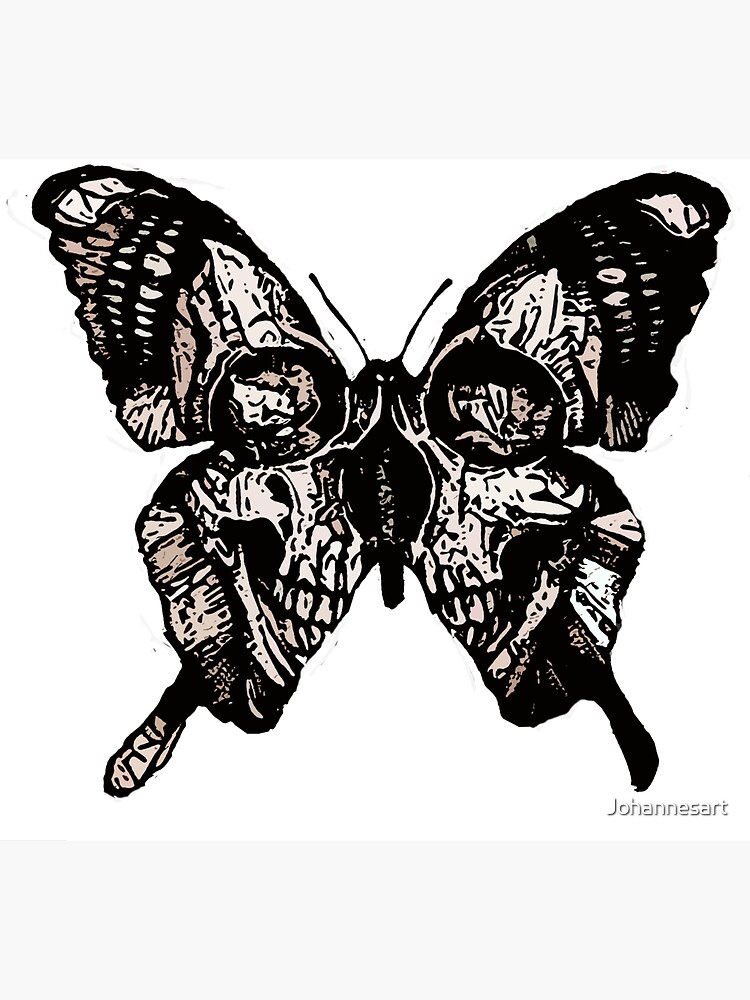This image is a detailed black-and-white drawing of a butterfly, reminiscent of eerie Mothman depictions. Set against a plain white background, the butterfly features intricate, unnerving patterns. The artist, Johan, has their credit inscribed in small block letters at the bottom right corner, "JOHANNESART." The butterfly's wings exhibit a blend of black, tan, off-white, and brown shades, with the black being more prominent toward the outer edges. The design includes negative space forming eye-like shapes near where the antennae, which extend upward and outward, meet the head. A skull appears subtly etched into the butterfly's back, contributing to its spooky aura. The wings showcase detailed patterns with varying shades and black circles near the body, creating a heavy contrast against the white background. This meticulous and chilling design seems purposefully crafted to evoke a sense of unease and fascination.